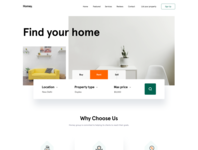The image displays a blurred screenshot of a website with a clean white background. At the top, there is a dark-colored print that is not legible due to the blurriness. Below the print, a horizontal menu bar spans from the middle to the right, containing six distinct words.

Below the menu bar, a square with unreadable text is present. Further down, the bold, large text "Find Your Home" appears prominently, with both 'F' in capitals. Beneath this text, two images are arranged side by side.

The left image is a smaller square depicting a minimalist room with a white wall adorned with mounted shelves. A bright yellow couch sits beneath the shelves, decorated with white and brown throw pillows, and it rests on a brown carpet.

The larger image on the right shows a room with an off-white to light gray wall. It includes a small table accompanied by a white plastic chair. A planter with a small plant is placed on the table. A banner with two white ends and a yellow or orange center stretches across the front of the table, containing text that is not specific in the description.

At the very bottom of the image, the phrase "Why Choose Us?" is displayed, completing the visual layout.